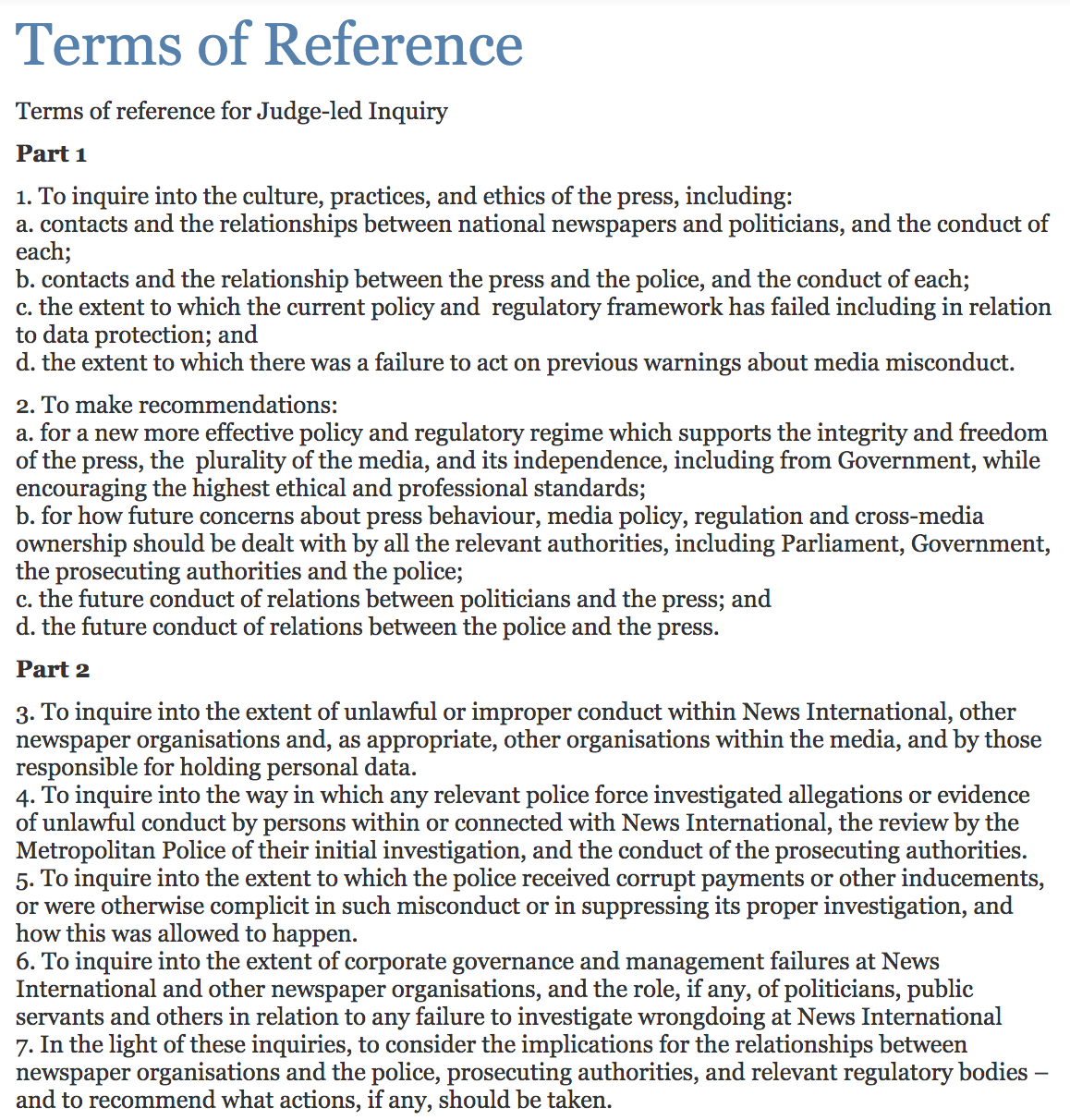**Descriptive Caption:**

The image displays an official documentation titled "Terms of Reference" in large, light blue font at the top left corner. Below the title, the subtitle reads "Terms of Reference for Judge-Led Inquiry," leading into the main content divided into multiple sections. 

**Part One** is introduced with bold formatting, outlining the scope "To inquire into the culture, practices, and ethics of the press, including," followed by an enumerated structure (A, B, C, D) that delves into various related subjects.

**Part Two** follows a similar format with a heading, stating "To make recommendations," and proceeds with points listed from A to D, akin to Part One.

Subsequently, **Part Three** initiates without splitting into subsections A to D. Instead, it enumerates continuous points, beginning with, "To inquire into the extent of unlawful or improper conduct within news, international, and other newspaper organizations, and as appropriate, other organizations within the media and by those responsible for holding personal data." This section continues through points four, five, six, and seven, maintaining a consistent format throughout.